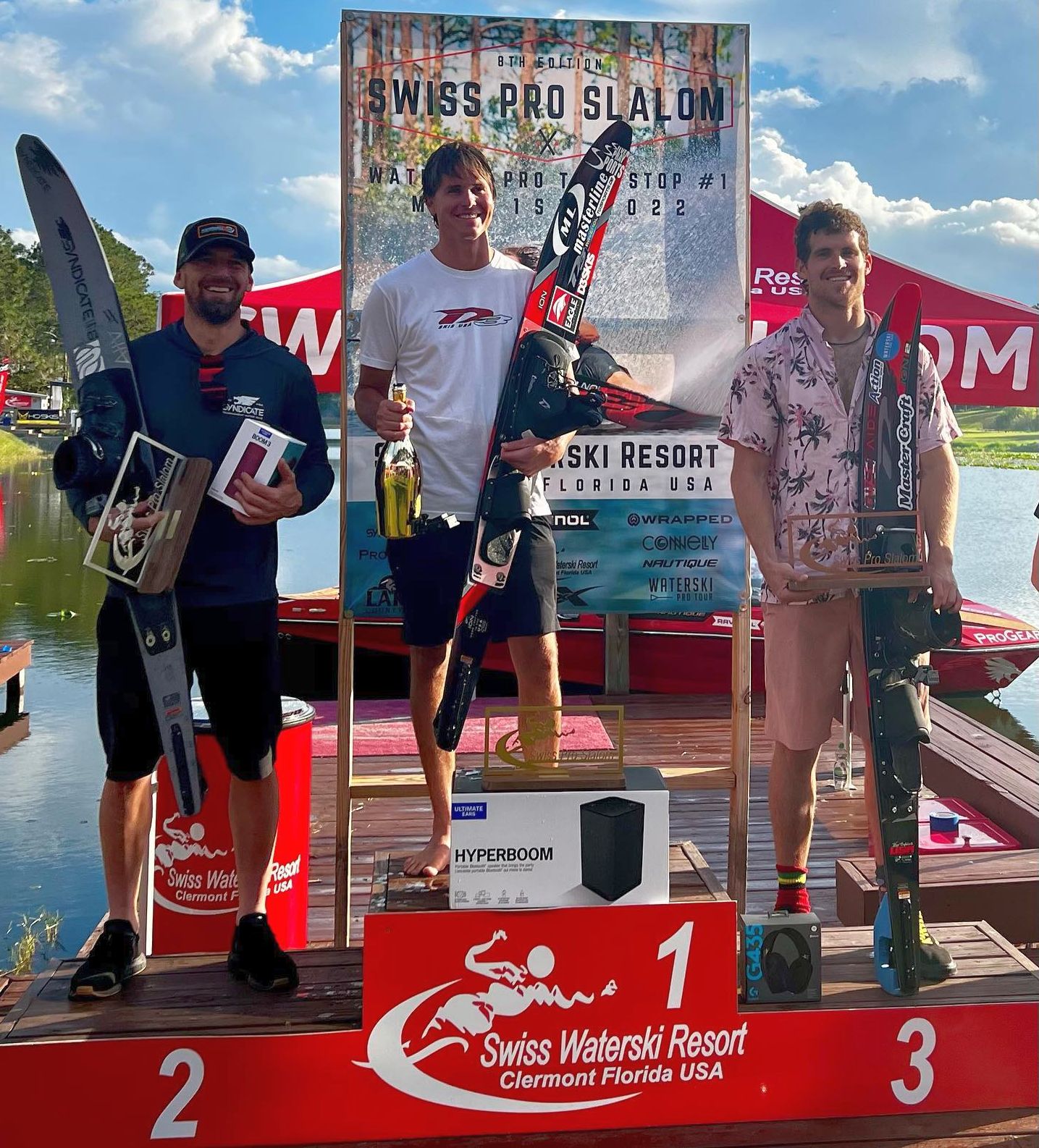The image captures a vibrant moment of victory at a water ski competition held at the Swiss Water Ski Resort in Claremont, Florida, USA. Three men are proudly standing on a podium with the numbers "1", "2", and "3" marking their respective places. The first-place winner is in the center, elevated on the highest part of the podium which is marked with a large number "1". He is dressed in a white short-sleeved shirt, black shorts, and is barefoot. In his right hand, he holds a bottle of champagne or wine, while his left hand grips a water ski. He has short dark hair and is beaming with joy.

To his left, on the second-place step marked "2", stands a man wearing a black hat, a blue long-sleeved shirt, black shorts, and black shoes. He is holding his water ski over his shoulder and balancing small boxes, his prizes, in his hands. On the right, occupying the third-place position marked "3", is another man dressed in a pink short-sleeved Hawaiian shirt, pink shorts, red socks, and black shoes. He too is holding his water ski along with his award.

Behind the trio, a large banner displays “8th Edition Swiss Pro Slalom,” with additional, partially visible text related to the competition. The background reveals a serene body of water and a red boat, under a sky filled with white clouds against a blue backdrop. The podium itself is inscribed with "Swiss Water Ski Resort, Claremont, Florida, USA" and features an image of a water skier, adding to the celebratory scene of this thrilling water sports event.